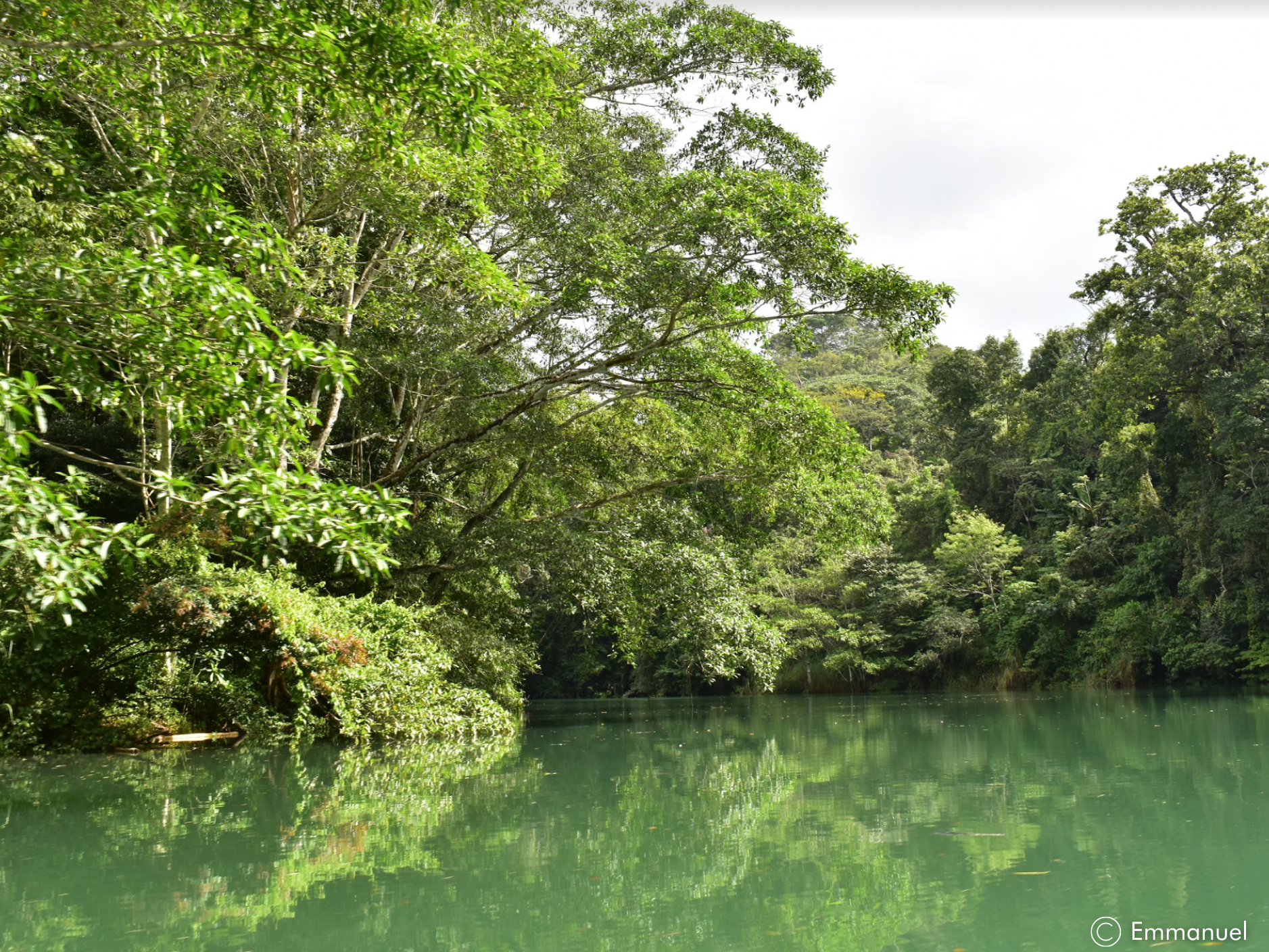This outdoor photograph, taken by Emmanuel, captures a serene and misty lake surrounded by an abundance of tall, healthy trees. The photo, taken in the daytime with plenty of daylight and clear skies, features a large bank of trees dominating the center and left of the image, their branches extending out over the still water. The surface of the lake is calm, reflecting the trees and branches, and small leaves float on the water. The sunlight, coming from the right side of the image, illuminates parts of the trees, indicating it is likely mid-afternoon. In the background, there is a dense grove of trees, creating a darker area that adds depth to the scene. At the bottom right corner of the image, a copyright mark spells out “Emmanuel.” There is some wood or possibly debris visible on the lower left bank of the water under the trees. The overall setting exudes tranquility with no visible boats, animals, or people.